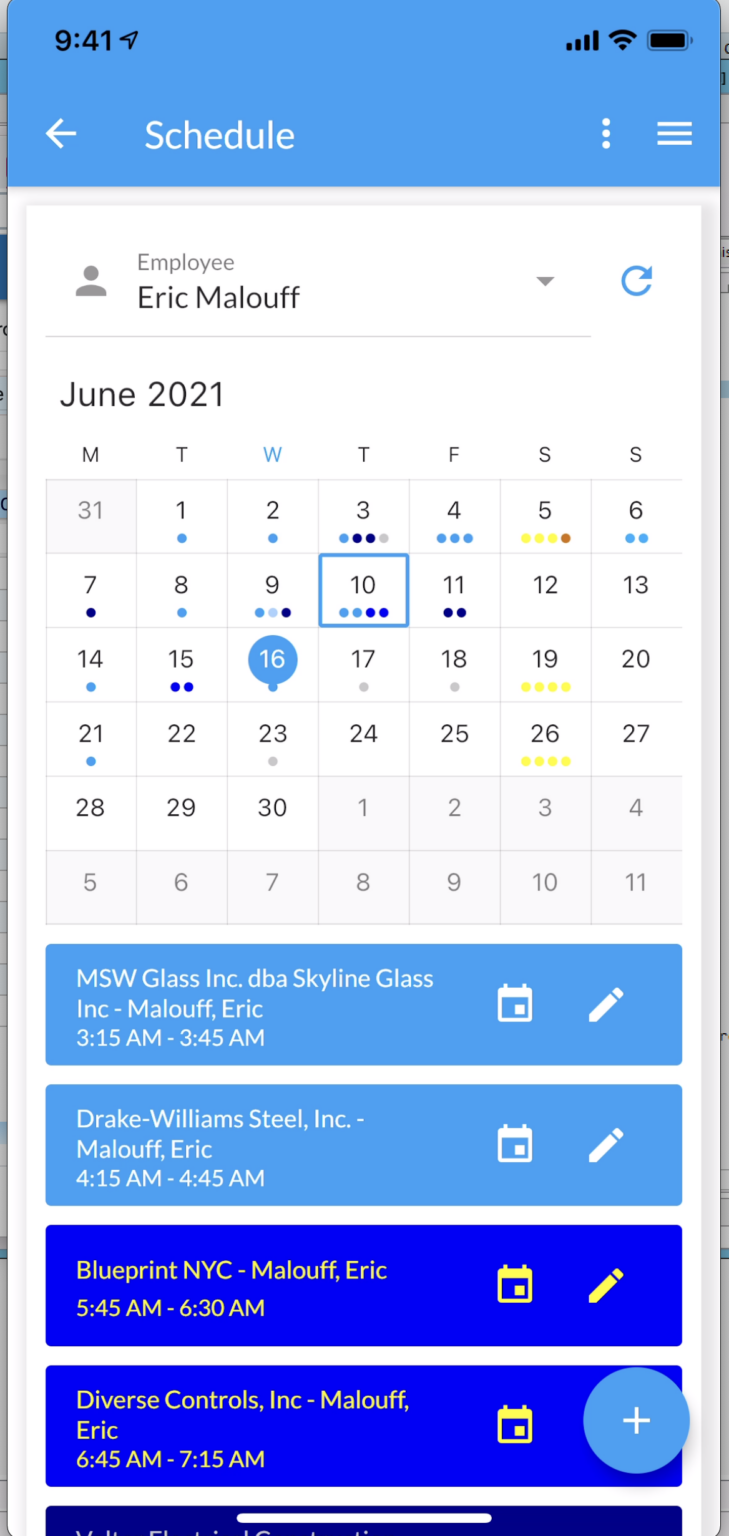A detailed screenshot of an iPhone digital calendar for June 2021, belonging to an employee named Eric Malouff, is displayed. The top section of the screenshot shows typical iPhone status indicators: the time in the upper left corner, and icons for Wi-Fi, battery life, internet connectivity, and phone signal strength in the upper right corner. Eric Malouff is identified as the user with a silhouette avatar, indicating no personal photo is attached.

The monthly calendar view highlights the dates June 10th and June 16th. Events for the selected dates are listed below. For June 16th:

- At 3:15 a.m., there is an entry for an MSW class.
- From 4:15 a.m. to 4:45 a.m., there’s an appointment with Drake William Steele.
- A scheduled event in a bold blue text box is listed as "Blueprint NYC" from 5:45 a.m. to 6:30 a.m.
- The final listing is a meeting with Diverse Controls Incorporated from 6:45 a.m. to 7:15 a.m.

Each entry represents various business meetings and commitments Eric has on this day.